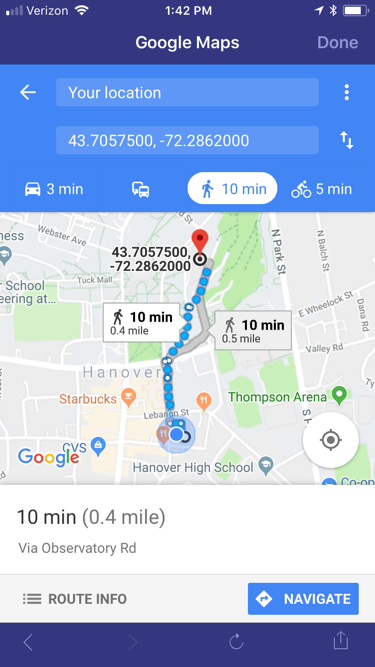This screenshot captures a Google Maps interface on a smartphone. At the very top, there's a blue bar displaying the standard phone status icons, followed by the title "Google Maps" prominently in white text. On the far right of this bar, a "Done" button is visible.

Directly beneath this bar, there's a lighter blue section containing two boxes. The first box indicates "Your Location," while the second box below it displays specific coordinates. To the right of these boxes, a series of icons show estimated travel times for different modes of transportation: car (3 minutes), bus (no time provided), walking (10 minutes), and biking (5 minutes).

Below this section, the main map area is displayed, featuring a red map pin towards the upper part of the screen, marking a specific location. The map also includes various routes and paths, denoting possible ways to reach the pinned location by the different travel methods indicated above.